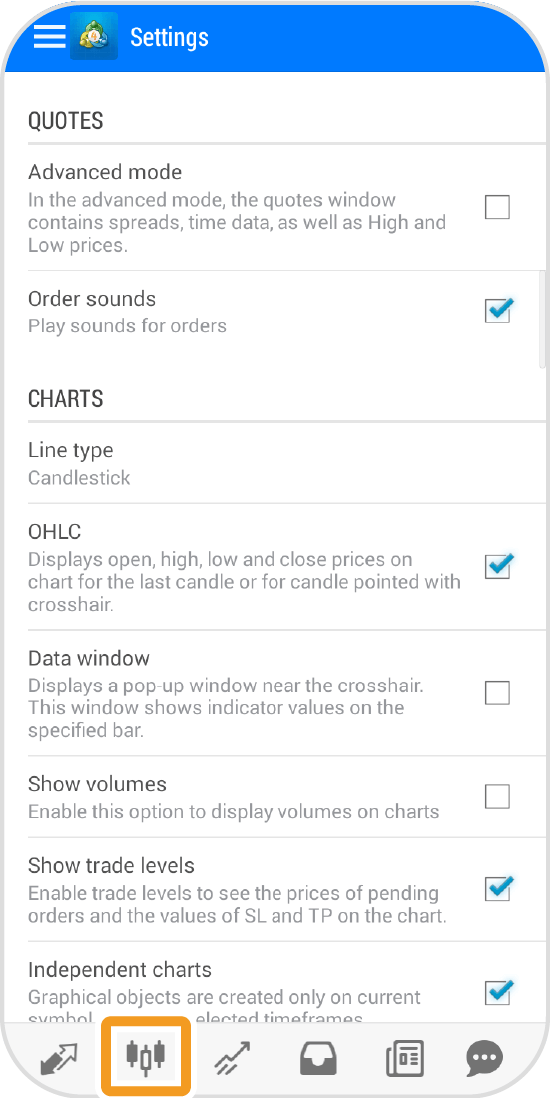The image appears to depict a settings screen from a mobile trading application. The layout is structured with a hierarchical menu format and features various trading parameters and customization options.

At the top of the screen, the title "Settings" is displayed prominently, accompanied by three horizontal menu bars. Adjacent to these bars, there is a small profile icon, predominantly blue, with an indiscernible symbol in the center.

Below the blue icon, the screen turns white, starting with a section labeled "Quotes" marked by a subtle gray line underneath. This is followed by the "Advanced Mode" option in black text. Within the Advanced Mode, the Quotes window offers detailed data such as spreads, time data, and high/low prices. There is an unchecked gray-outlined box next to this option.

Continuing down, a fine gray line separates the following item: "Order Sounds" in black text with the subtext "Place Sounds for Orders." This option is activated, indicated by a blue-checked box.

Next is the "Charts" section, again separated by a fine gray line. This contains the "Line Type" option, set to "Candlestick." Another fine gray line precedes the "OHLC" setting, displaying "Open, High, Low, and Close Prices on Chart for the Last Candle, or for Candle Pointed with Crosshair," which is also enabled, denoted by a blue check mark.

Below this, the "Data Window" option is mentioned in black, explaining that it displays a pop-up window near the crosshair to show indicator values per specified bar. This box is not selected.

Following another fine gray line, the "Show Volumes" option is present, meant to enable volume display on charts; this setting is unselected.

The "Show Trade Levels" setting is next, explaining it allows the display of pending orders and SL/TP values on the chart. This option is checked in blue.

Near the bottom, the "Independent Charts" option is described, stating that graphical objects are created only on the current symbol. This option is also enabled, as denoted by the blue check mark, though some of the text gets cut off due to a bottom banner on the screen.

At the very bottom, there are navigational icons: a solid black down arrow alongside a white-up arrow outlined in black. Additionally, there's an orange-outlined box containing three small icons: a black icon on the left, a white icon with a black outline in the middle, and a black icon on the right. The rightmost icon features an upward-pointing arrow.

Further icons include a small square with a white top and black bottom, a black outline of a square with horizontal lines, and a black chat icon with three white dots.

Overall, the detailed description of the settings screen emphasizes the customization and functionality options available for a trading app user.